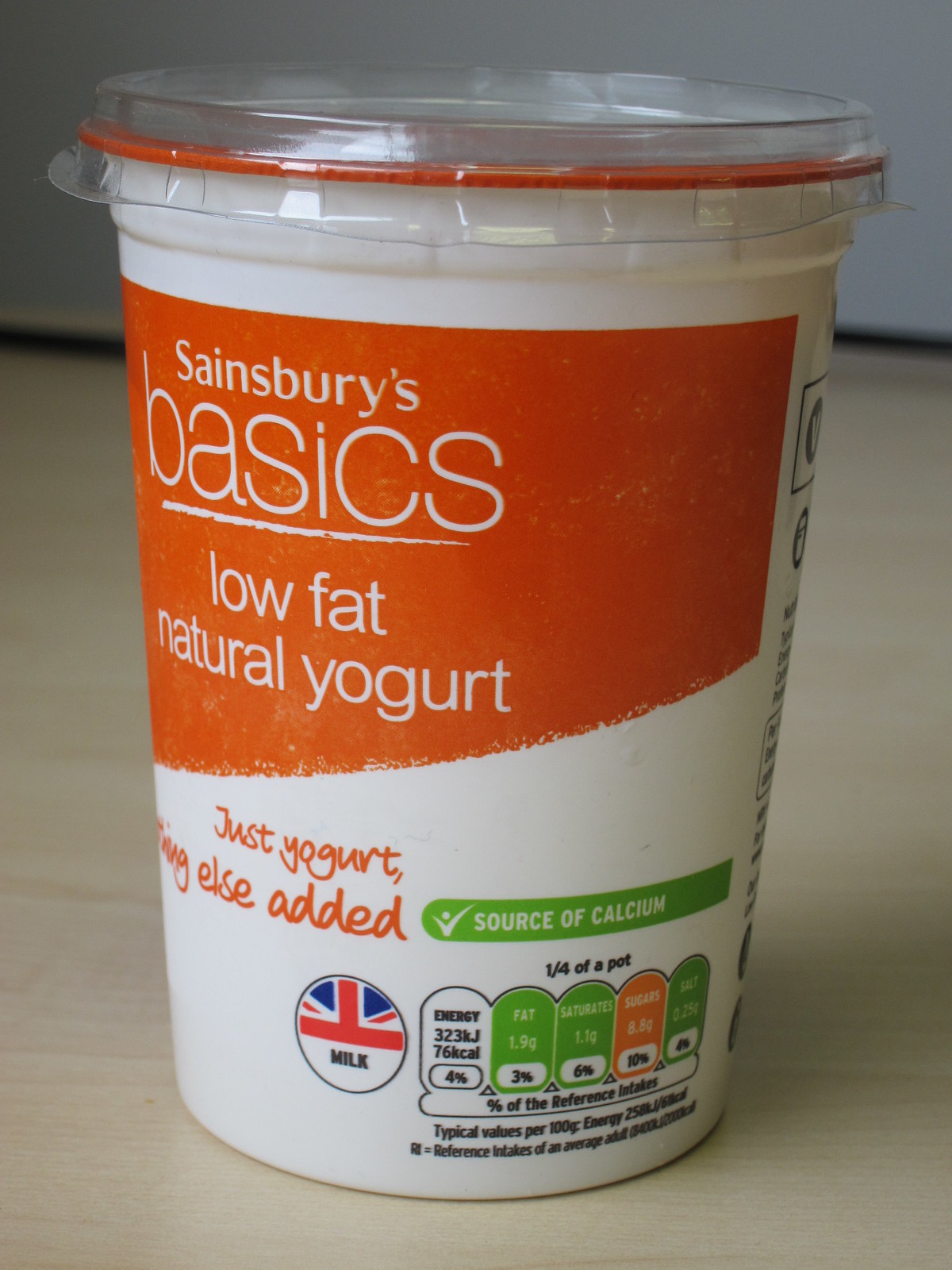This photograph showcases a plastic container of Sainsbury's Basics Low Fat Natural Yogurt, positioned on a light wooden table against a white wall. The white container features a prominent orange banner at the top, which states "Sainsbury's Basics Low Fat Natural Yogurt" in white lettering. Below this, in an orange script, the phrase "just yogurt, nothing else added" is visible. Adjacent to this, a green banner proclaims it as a "source of calcium." Further down, in a partially white section, detailed nutritional information is listed: 1/4 of a pot provides 323 kJ (76 kcal), 4% energy, 1.9 grams of fat (3%), 1.1 grams of saturates (6%), 8.8 grams of sugars (10%), and 0.25 grams of salt (4%). Additionally, part of the Union Jack is displayed in a circular design, indicating the product's UK origin, with the word "milk" printed below it in black letters. The clear plastic lid completes the minimalist yet informative presentation of this yogurt container.